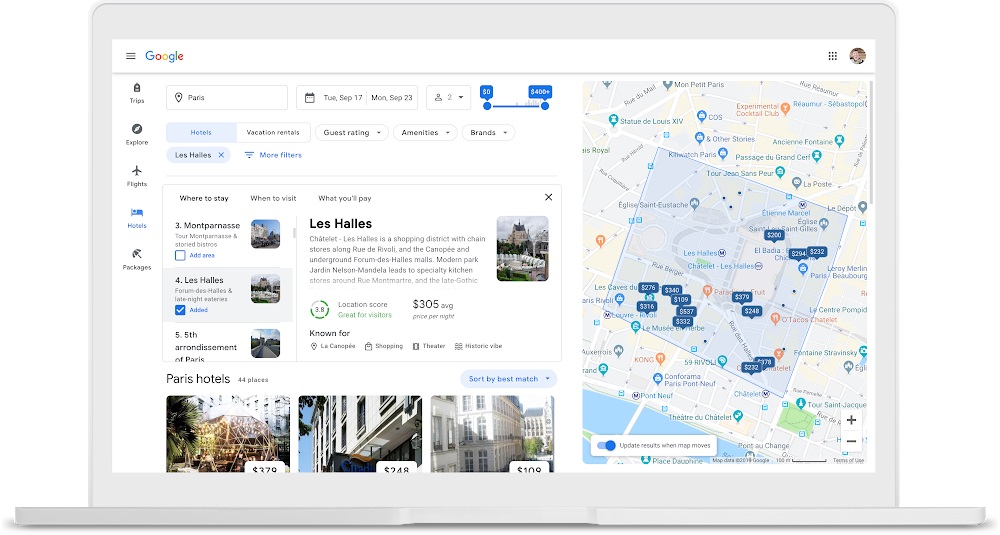The image, set against a pristine white background, features a sleek, white monitor or possibly a tablet displaying a detailed screenshot of a Google search result. In the upper left corner of the screen, the recognizable Google logo is visible. To the right, there is a circular icon containing an illustration of a man’s face and shirt. Below this, the text "Paris" appears in the upper left corner, followed by navigation options: Trips, Explore, Flights, Hotels, and Packages, with the "Hotels" tab highlighted.

The search query results indicate specific dates from Tuesday, September 17th through Monday, September 23rd, for two people. The list of hotels provides detailed information with rankings, starting with number three, Montparnasse; number four, Les Halles; and number five, the Fifth Arrondissement of Paris. To the right, more details about Les Halles are displayed, including the average cost per night at $305, and a location score of 3.8, noted as "great for visitors."